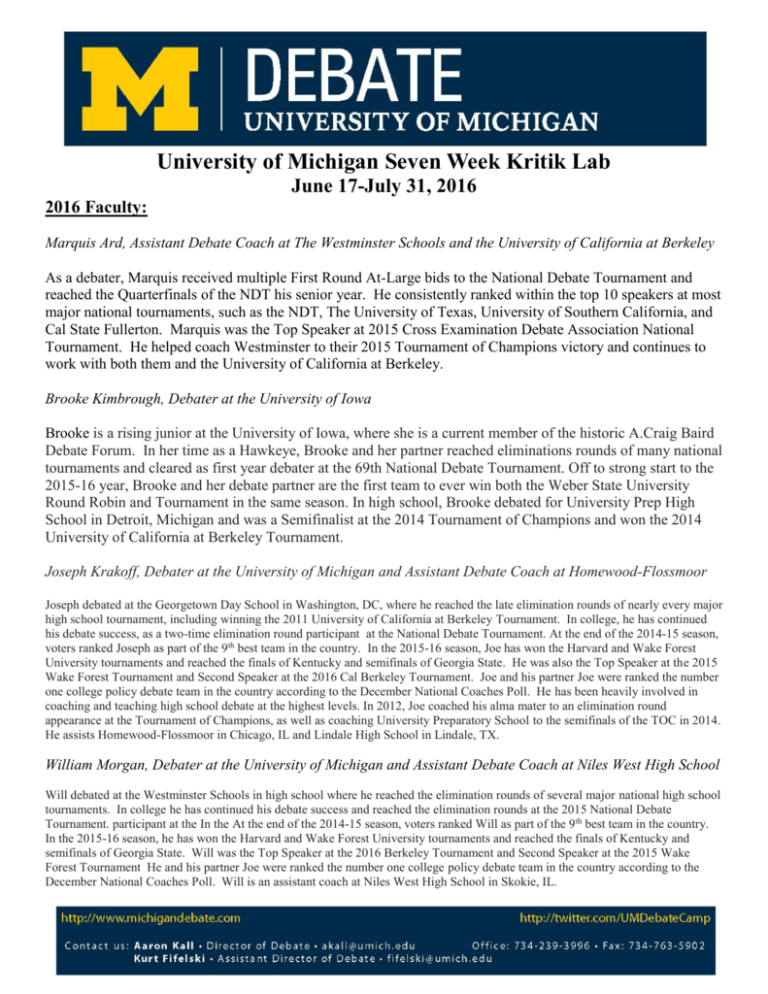The image is a screenshot of an article from the University of Michigan website, specifically related to their debate program. A prominent dark blue banner spans the top of the page, displaying the iconic large yellow "M" logo. Beside the logo, text in white reads "Debate University of Michigan." Directly beneath that, in black text, it states "University of Michigan Seven Week Critic Lab, June 17th to July 31st, 2016."

The title "2016 Faculty" follows in bold, underlined black text. Below this title, there are several sections, each with introductions for different faculty members participating in the lab. The first section is marked with an italicized heading, presenting Marquess Art, Assistant Debate Coach at The Westminster Schools and the University of California at Berkeley. A brief paragraph provides additional details about Marquess Art.

Next is Brooke Kimbrough, a debater at the University of Iowa, followed by Joseph Krakow, a debater at the University of Michigan and Assistant Debate Coach at Homewood-Flossmoor. Joseph Krakow has the most extensive write-up among the faculty members. Lastly, William Morgan is introduced as a debater at the University of Michigan and Assistant Debate Coach at Niles West High School, with a descriptive paragraph about him as well.

At the bottom of the page, another dark blue banner appears. It lists a website and a Twitter address in gold text, along with contact information for Aaron Kall, the Director of Debate, and Kurt Fifelski, the Assistant Director of Debate. Email addresses, an office number, and a fax number are provided for each.